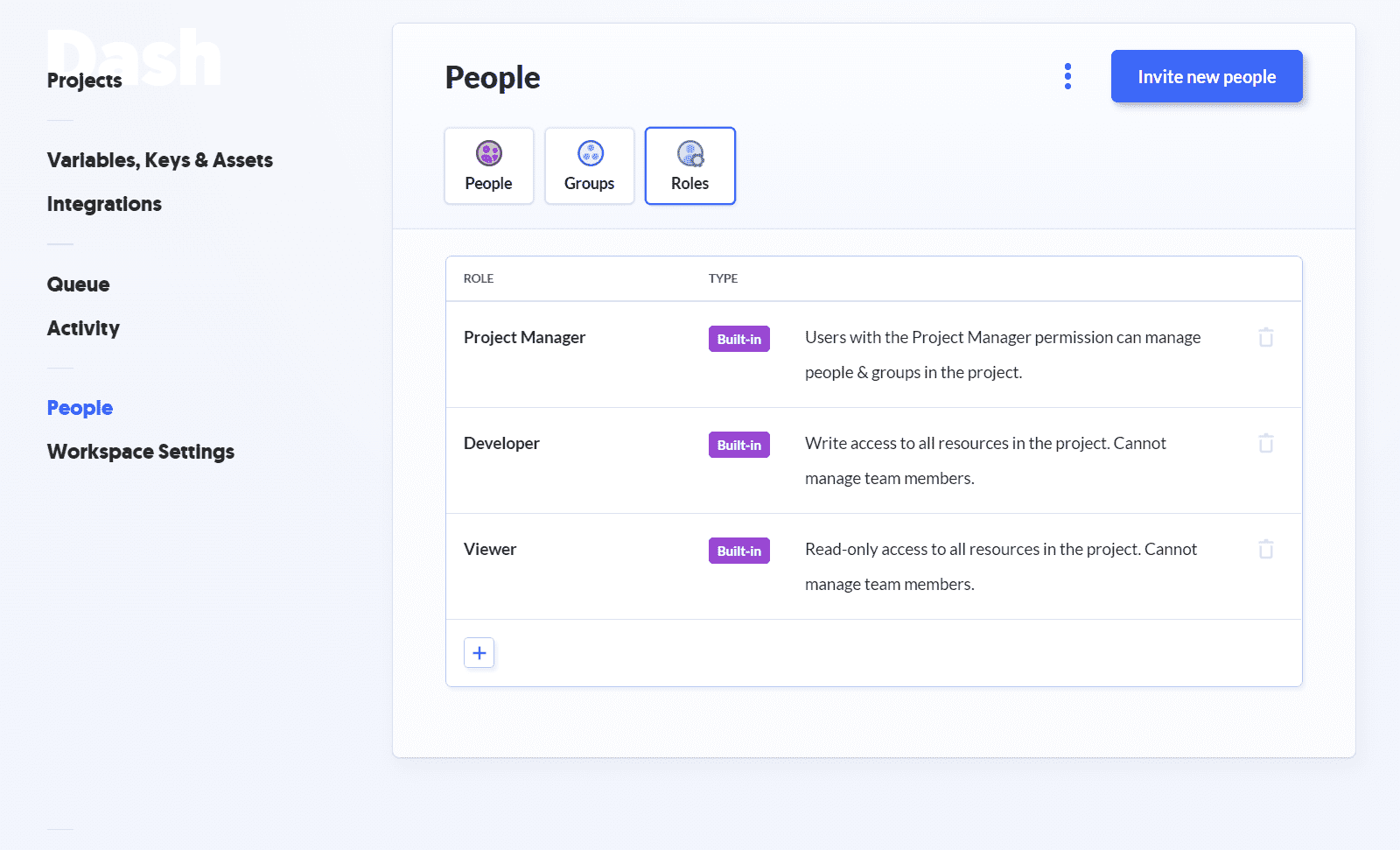**Detailed Caption:**

The image showcases a settings page for an application or website named "Dash." The interface is titled "Dash Projects," set against a light gray or light blue background with black text, accented in shades of purple and blue. On the left side, a vertical menu displays several options: Variables, Keys and Assets, Integration, Queue, Activity, People (highlighted in blue as the current selection), and Workspace Settings.

To the right, there's a pop-up window titled "People." Within this window are three tab buttons labeled People, Groups, and Roles, presumably to filter users by different categories. Additional options are presented via a vertical ellipsis menu, along with a prominent blue button with white text labeled "Invite New People."

Below this interface, there's a table formatted into two columns: Roles and Types. The Roles column lists three user categories—Product Manager, Developer, and Viewer—while the Types column consistently reads "Built-in." Detailed descriptions specify the permissions associated with each role. The Product Manager is granted permissions to manage people and groups within the project. Developers have write access to all resources but cannot manage team members. Viewers are limited to read-only access to resources and are also unable to manage team members.